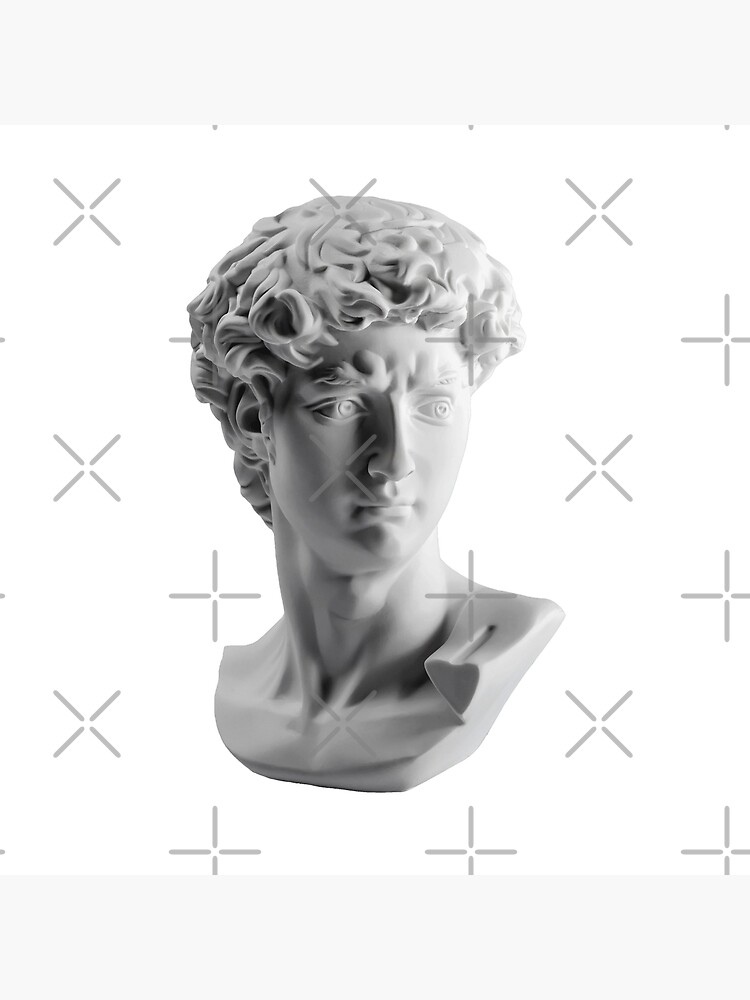The image features a detailed bust sculpture of Michelangelo's David, prominently displaying the head, neck, and partial shoulders. The man depicted in the bust has a worried or irate expression, characterized by furrowing eyebrows and tightly knit wrinkles, as he looks towards his left (right from the viewer's perspective). The sculpture is made from greyish stone, with a smooth surface and subtly wavy hair. The bust is placed directly at the center of the image. The background is white, adorned with light grey X and plus shapes that resemble watermarks, some of which overlap the sculpture. There are also two grey patches at the top and bottom of the image. The style and setting evoke the appearance of an ancient Greek or Roman sculpture.